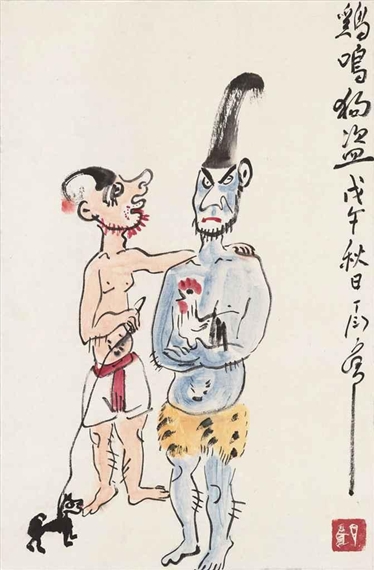The image is a highly stylized, cartoonish drawing of two humanoid creatures against a light blue background. On the left stands a pale-skinned figure, shirtless with white shorts detailed by red horizontal and vertical stripes. This figure sports a sparse red beard and a curved hat with a red pom-pom. In his hand, he holds a leash attached to a black dog. The character on the right is bluish-skinned with a pronounced angry red frown and a black beard. He wears tan, spotted shorts resembling animal fur and cradles a chicken in his arms. His hat, tall and slightly curved to the right, further accentuates his intense expression. A red signature is present at the bottom of the image, and there is text in Chinese characters along the right edge.